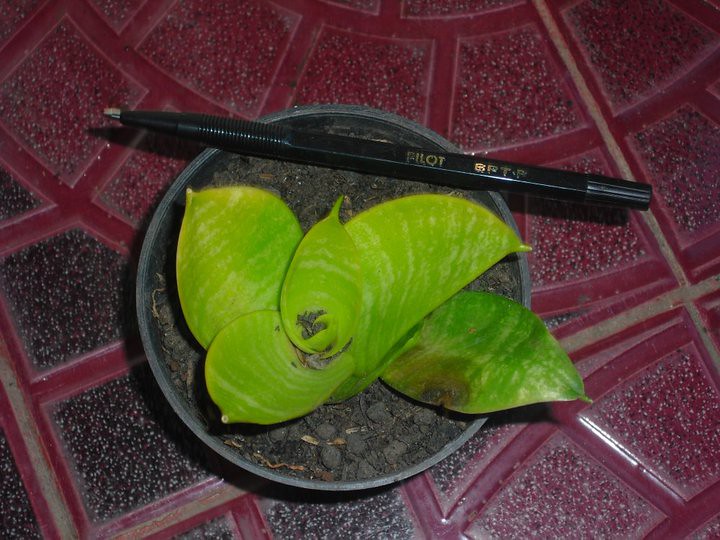This is a detailed, top-down, color photograph in landscape orientation. The main subject is a small green plant with five leaves, four on the sides and one in the center, growing in a round gray pot filled with dark brown, slightly dry soil. A black pen, resting diagonally from the top left to mid-right of the pot, provides a sense of scale for the plant and container. The pot is placed on a distinctive radial patterned floor composed of dark pink and black tiles in a circular arrangement, resembling linoleum. The entire scene is devoid of any human elements, dates, or additional plants, capturing a solitary and serene atmosphere.